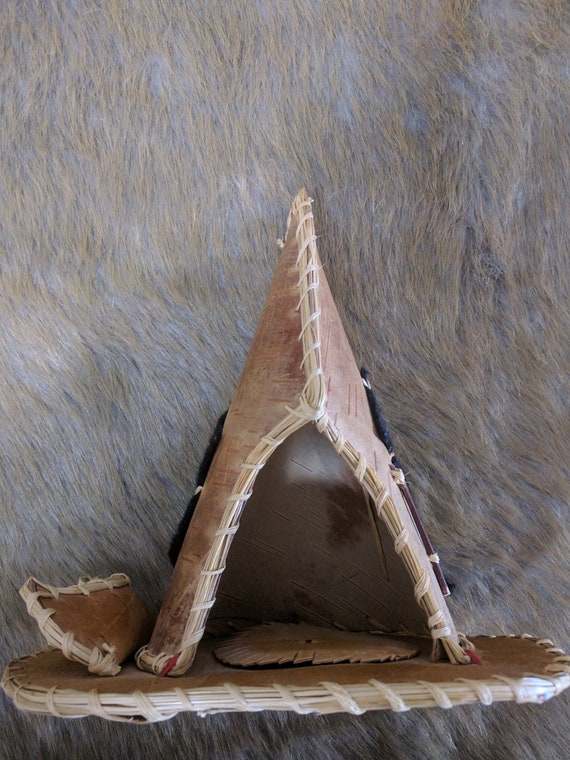The image features a detailed, miniature Native American display centered on a handcrafted teepee and related artifacts. The teepee, made from light brown canvas with black vertical stripes, is intricately stitched with white string along its edges. It sits on a base of light brown leather, approximately four inches long and oval-shaped. The teepee's opening faces the camera, revealing a white, round object inside, perhaps mimicking a rug. The backdrop is a luxurious, fur-like surface in shades of light brown to gray, possibly intended to evoke natural animal hides. Adjacent to the teepee is a small, brown leather canoe, also adorned with white stitching, tilted on its side. The overall color palette of the display includes earthy neutrals: black, white, brown, gray, and tan. This meticulously arranged scene, devoid of text or human presence, appears designed for educational purposes or a detailed catalog, with studio lighting accentuating its elements against the fur background.